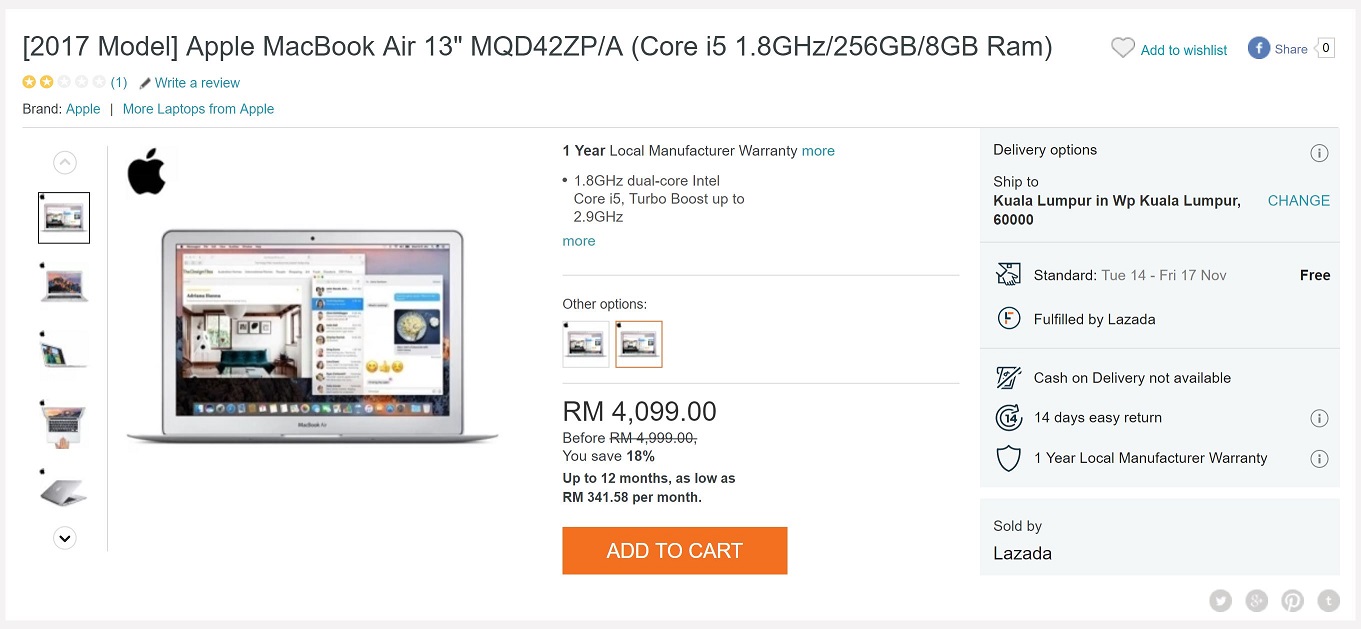A detailed screenshot of a webpage displaying the listing for a "2017 Model Apple MacBook Air, 13-inch, MQD42ZP/A." The layout is horizontally oriented with a white background and black text predominantly concentrated in the upper left and across the top. The top text details the model and specifications of the product. Below that is an image of the laptop, which displays an open screen showcasing a room with a sofa and several emojis. The iconic Apple symbol is visible in the top-left corner of the laptop's screen.

Adjacent to the image, a block of text provides further details: "One year local manufacturer warranty." Below this, the price is listed, and an orange "Add to Cart" button is prominently positioned in the lower center of the page.

On the right side, shipping details are highlighted: "Delivery options, Ship to Kuala Lumpur and WP Kuala Lumpur." Additional information includes: "Standard Free Fulfilled by Lazada," "Cash on Delivery Not Available," "14 Days Easy Return," and "One Year Local Manufacturer Warranty Sold by Lazada." The overall context suggests that this webpage is facilitating the purchase of a pre-owned Apple MacBook Air, clearly presenting the product details, price, warranty, and shipping information.